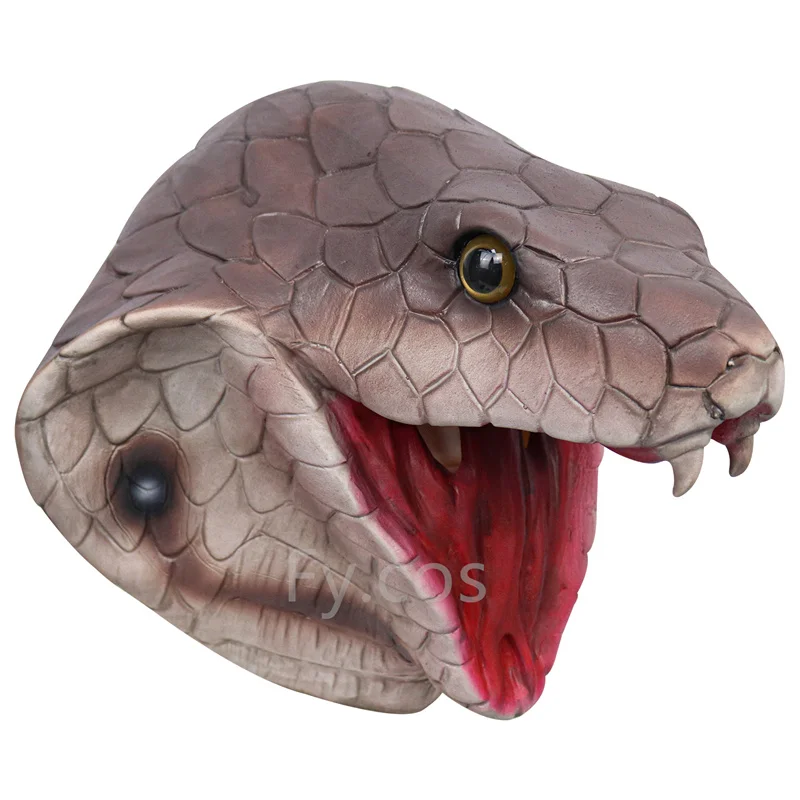The image depicts a close-up of what appears to be a rubber or animatronic replica of a rattlesnake's head set against a white background. The snake's head is oriented slightly forward and to the right, with the nose visible on the right side. The coloration transitions from a darker gray at the top of the head to lighter hues towards the bottom of the mouth and neck. A yellow eye with a black pupil stares slightly off-center towards the camera. The snake's mouth is wide open, revealing a pink, forked tongue and a pink mouth interior, and exposing two sharp fangs at the upper tip of the mouth. There is a small gray, white, and black dot at the neck, possibly a fastening section. A watermark that reads "FY.COS" is visible on the image, indicating the source of the photograph.